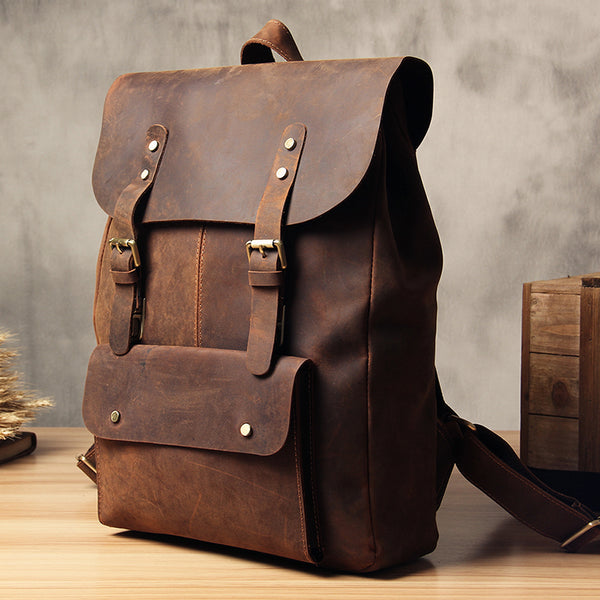This professionally taken photograph features a weathered brown leather backpack or messenger bag, standing upright on a light-colored wooden table. The backpack, crafted from oiled and slightly cuffed leather with lighter patches, is taller than it is wide and showcases a classic, traditional design. The bag has a large top flap secured with two buckle straps, and a smaller rectangular pouch on the lower front with a flap closed by two metal snaps. A small brown leather loop at the top allows the backpack to be hung on a hook. Part of the backpack's carrying straps is visible, jutting off to the sides. The background includes a mottled gray wall, a wooden box to the right, and what appears to be the end of a broom resting on a book to the left.